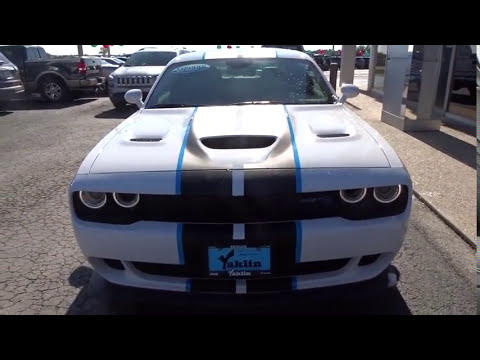In this daytime photograph, a white Dodge Challenger with distinctive black racing stripes, bordered by thin light blue lines, takes center stage in an outdoor setting at the Yaklin car dealership. The Challenger features four prominent headlights, two on each side, and multiple vents, including a large scoop in the center of its hood. The car is parked on a gray asphalt surface with visible cracks, and a price tag is attached to its windshield. The dealership name, "Yaklin," is visible on a light blue license plate holder at the front of the car. Surrounding the Challenger are various other vehicles, including a Jeep Grand Cherokee and a truck, also parked and ready for sale. In the background, the dealership building can be seen on the right, characterized by its glass windows and concrete pillars.